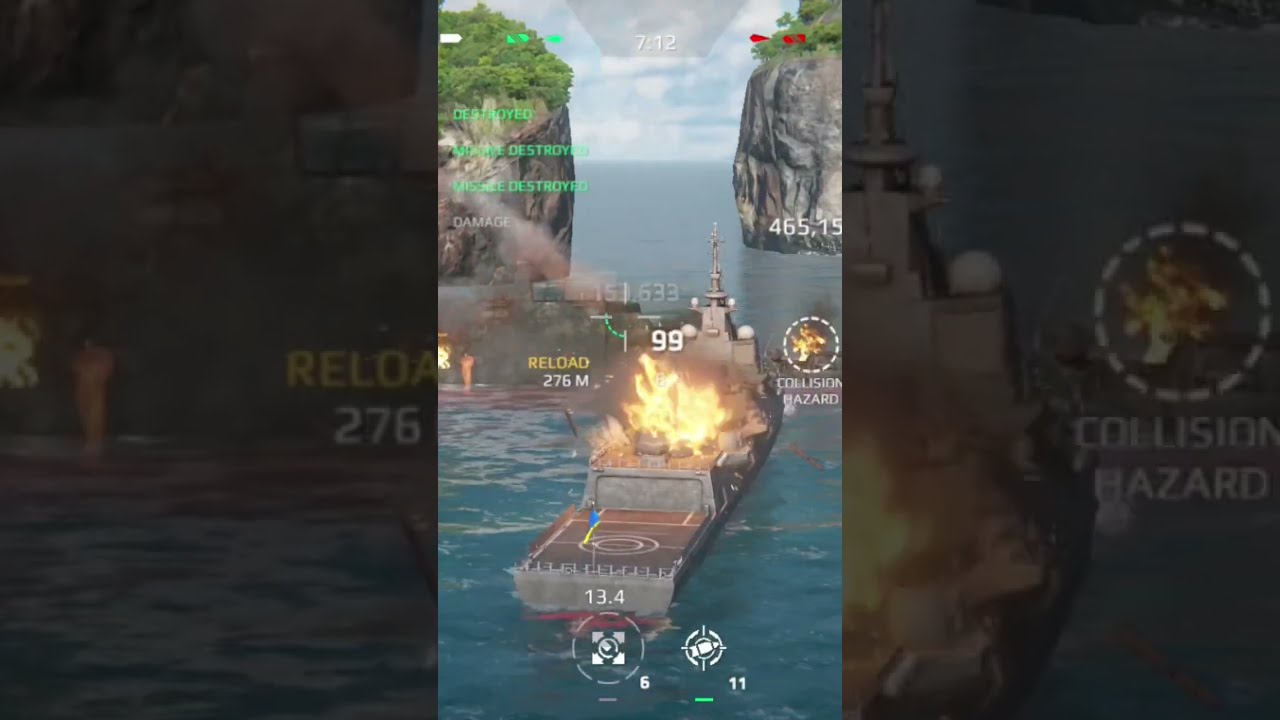The image is a detailed screenshot from a 3D mobile warship or battle game. The central focus is a modern destroyer warship, currently on fire following a missile hit to its superstructure. The warship is navigating through a water passage flanked by two steep, rocky cliffs with green, bushy plateaus on top. The water beneath the ship transitions from turquoise to blue towards the horizon. UI elements are prominently displayed: at the bottom, there are controls and damage indicators, including symbols with the numbers 6 and 11, and a bar indicating active play. The left side of the central image shows a magnified and darkened view of the "reload 276 mil" text, while the right side highlights the explosion on the destroyer with the number 99 above it and a "collision hazard" symbol nearby. At the top, clouds hover above the water with the time "7:12" or "742" visible, and there are red symbols to the right. The left cliff features some small white rectangles and green lettering, adding to the game's immersive environment. The entire image is framed by an enlarged, darkened version of the central screenshot, enhancing the dramatic effect of the active battle scene.